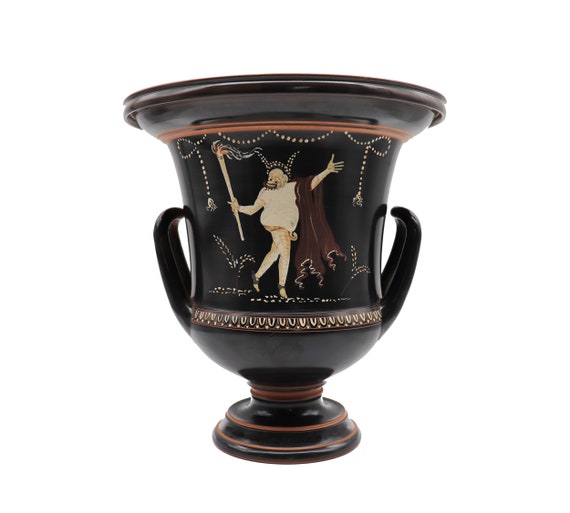The image depicts a glossy black trophy-like cup set against a white background. The cup has an intricate design featuring a central figure, reminiscent of a mythical creature or human, draped in a white robe with a brown shawl over its left arm, and holding a staff or torch in its right hand. This figure appears to be surrounded by what looks like trees or vines. The cup itself is large at the top and tapers down to a narrower base, which consists of two circular levels - an orange accented lower base and a smaller, concentric top level. The cup also features two curved black handles that attach to the cup at the bottom but not at the top, forming an open arc. The overall colors of the design are black, gold, orange, and brown, and no text or numbers are visible on the cup.